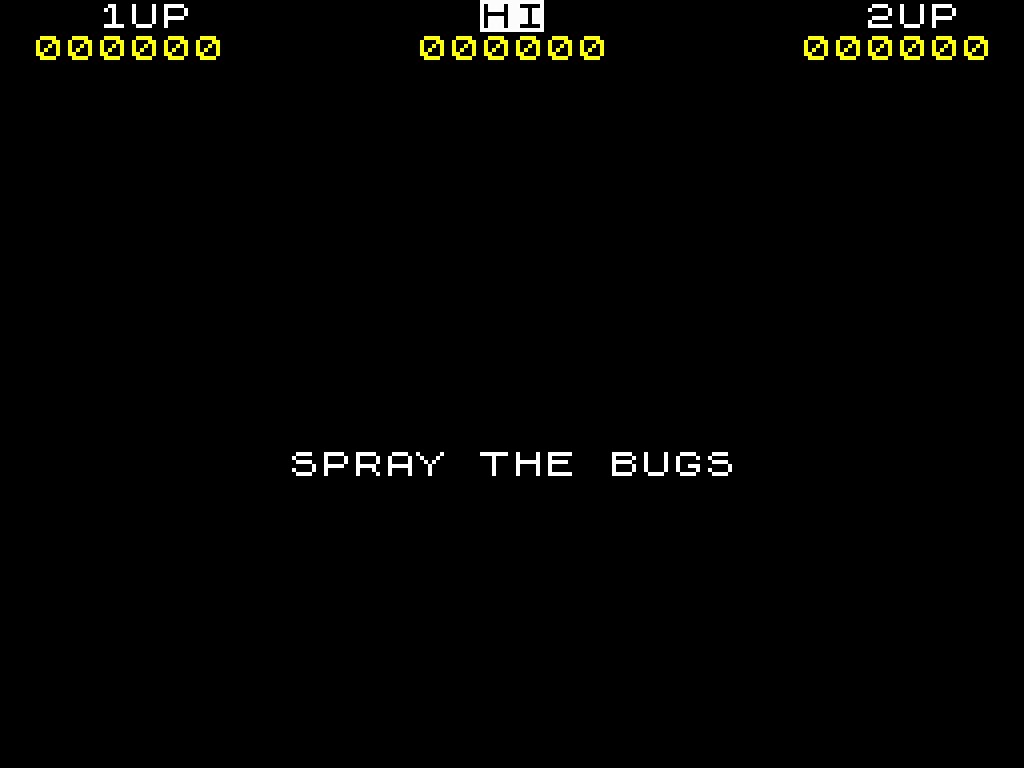This image is a screenshot from a video game interface. The screen is predominantly black, with several colored elements. In the top left corner, there is white text that reads "1 UP," and directly below it in yellow text, the score displays as "000000." Centered on the screen is a white rectangle with the word "HI" in black letters inside it. Underneath this, in yellow text, another score reads "000000." In the top right corner, white text reads "2 UP," with a yellow score of "000000" directly below it. Across the middle of the screen, bold white capital letters command, "SPRAY THE BUGS."